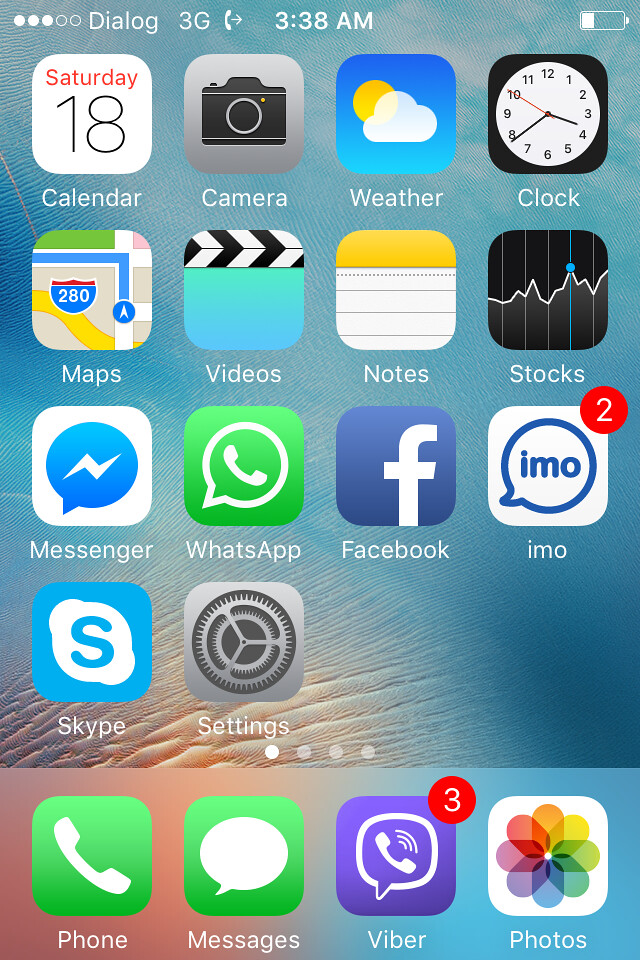A detailed screenshot of a smartphone screen captures a moment in time at precisely 3:38 AM. The status bar at the top of the screen shows various indicators: the 3G network symbol, three out of five filled circles indicating signal strength, a battery icon representing low battery life, and a small phone and arrow icon suggesting some form of call activity or notification. The visual backdrop of the phone features an elegant, serene image reminiscent of a coastal scene with light blue and tan hues mimicking water and sand under the sky.

Prominently featured is an app calendar icon marked with the date "18th Saturday" in a clean, white box. An array of well-organized app icons is displayed, including the camera, weather, clock, maps, videos, notes, stocks, messenger, and WhatsApp (distinguished by its green icon). Additionally, Facebook is represented with its familiar blue logo, IMO with an indication of two unread messages, Skype, and settings complete this app selection.

On the bottom banner of the screen, a neatly arranged row of essential apps is shown. From left to right, there is a phone icon for dialing, messages with an accompanying indication of three unread messages signified by a red circle, the Viber app characterized by its purple icon featuring a white phone inside a speech bubble, and lastly, the gallery photos app. This captivating screenshot intricately details the smartphone interface and provides a snapshot of the user's digital environment.